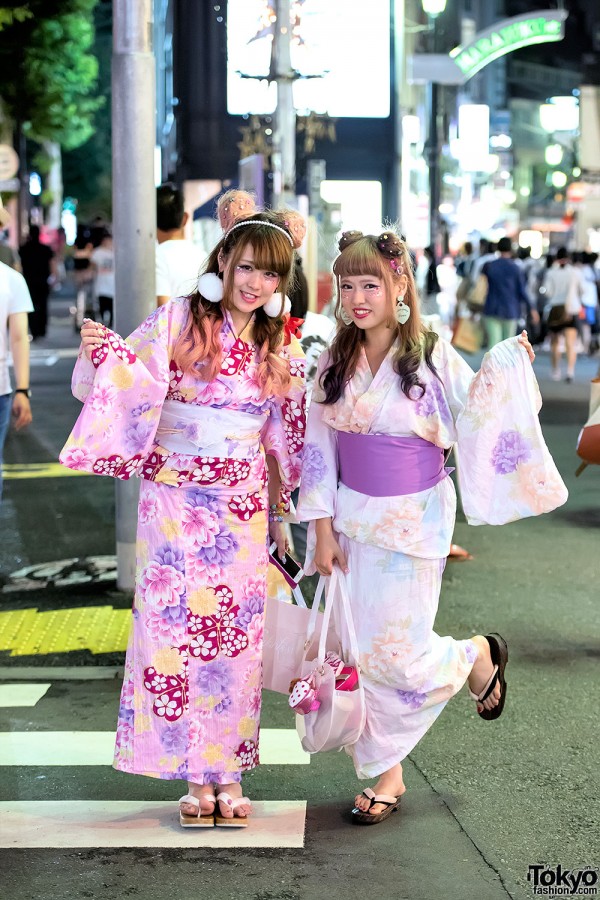This image depicts a busy intersection in Tokyo, Japan, where two women dressed in traditional Japanese kimonos are posing in a pedestrian crosswalk. The bustling background features blurred people and a streetlight pole, suggesting a vibrant urban setting. These women appear to be the focus of a professionally taken photograph, possibly for a magazine, as indicated by the "tokyofashion.com" watermark in the lower right corner.

The woman on the left has long brunette hair with pink tips and adorns white puffball earrings. She wears an exquisite pink kimono, intricately decorated with floral patterns in shades of light pink, purple, yellow, and dark pink. Her kimono boasts the characteristic long sleeves of traditional attire, and she completes her outfit with white flip-flops.

Beside her, the woman on the right, who has blonde hair with brunette tips styled in two buns, holds a heart-shaped purse accessorized with a cupcake keychain. She is dressed in a light white kimono adorned with delicate purple and beige flowers, and it is cinched with a purple sash. Her ensemble is finished with matching flip-flops and heart-shaped earrings. The lively atmosphere of the Tokyo street scene, coupled with their elegant traditional clothing, creates a striking and culturally rich visual.